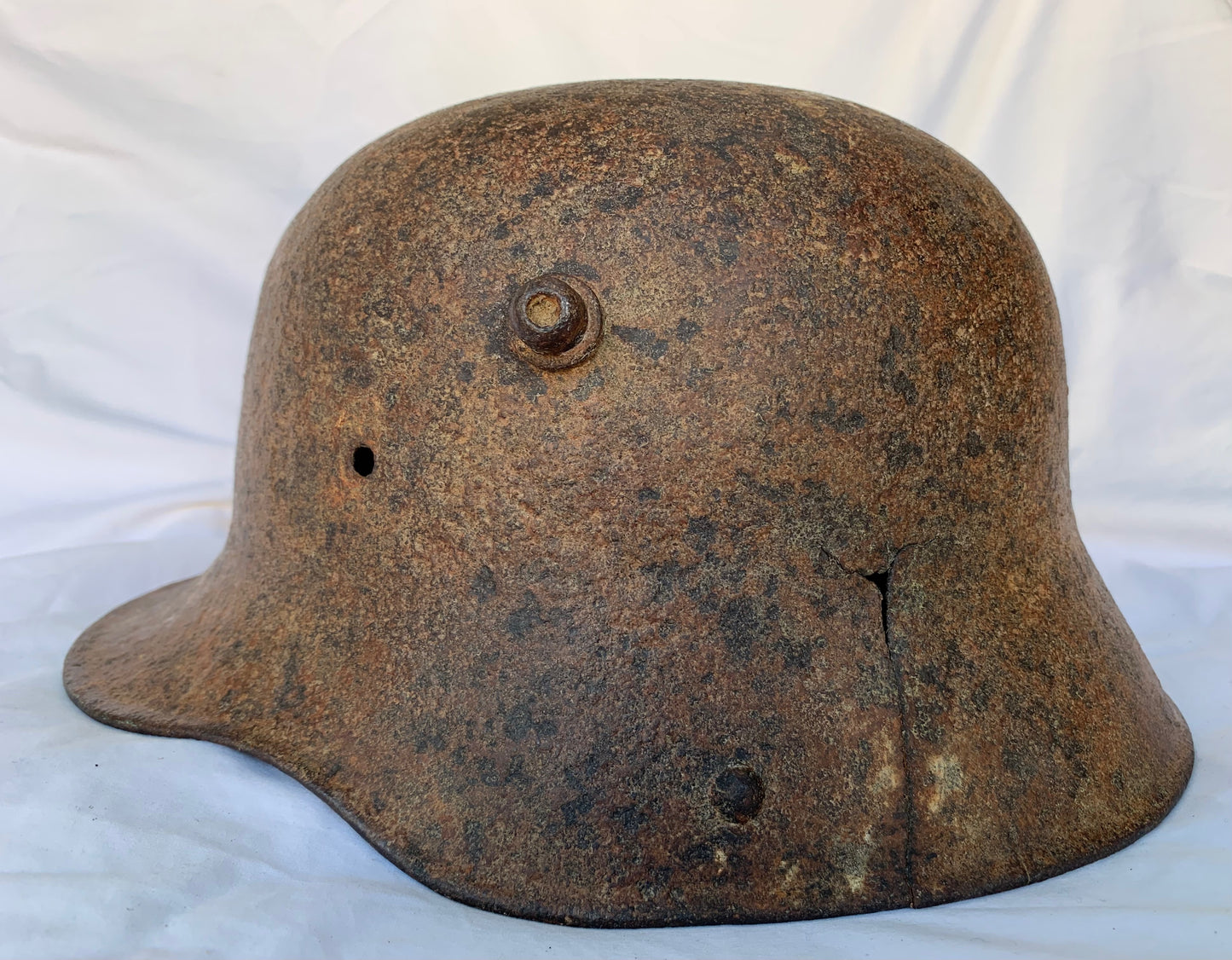This photograph showcases a heavily rusted German army helmet, positioned on a white sheet that creates a shaded foreground. The well-lit image details the helmet's decrepit state, with the original finish almost entirely gone, replaced by a predominantly brown and black rusted exterior. The dome-shaped, steel helmet, viewed from a three-quarter angle, reveals significant damage: a prominent crack runs up the back and a potential bullet hole near the ear. Additional features include a heavily corroded nut likely used to attach headgear and speckled black inserts. This helmet, possibly dug up after many years exposed to the elements, offers historical value despite its dilapidated condition.